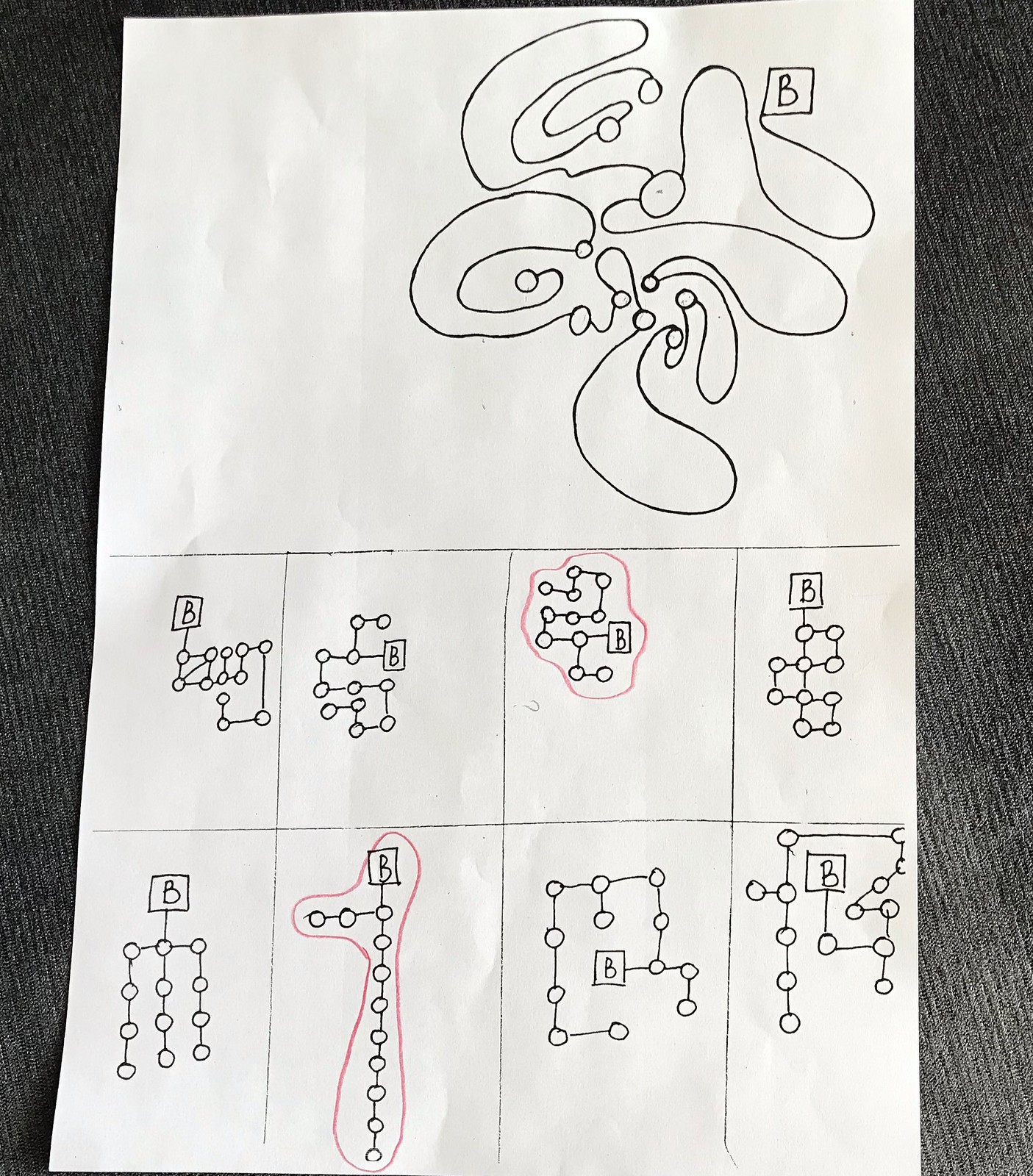This indoor, close-up color photograph features a piece of paper lying vertically on a tan, low-pile carpet, visible on both the left and right sides of the image. The paper contains intricate, deliberate patterns rather than casual doodles. In the upper right corner, a collection of dots is connected by aged lines, and adjacent to it, there is a small square with the letter "B" inside.

The bottom half of the paper is segmented into two rows of four rectangles each. Within each rectangle is a distinct arrangement of dots, connected by horizontal and vertical lines, along with a small square containing the letter "B" in various positions. The patterns within these rectangles are meticulously drawn, suggesting a structured sequence or molecular pattern.

Notably, in the top row, the third rectangle from the left has been circled in red pen, and in the bottom row, the second rectangle from the left is similarly circled. The dots in the bottom row form vertical columns, further indicating a purposeful design rather than random doodling. This paper likely represents a specific sequence or pattern, possibly of scientific or mathematical relevance.